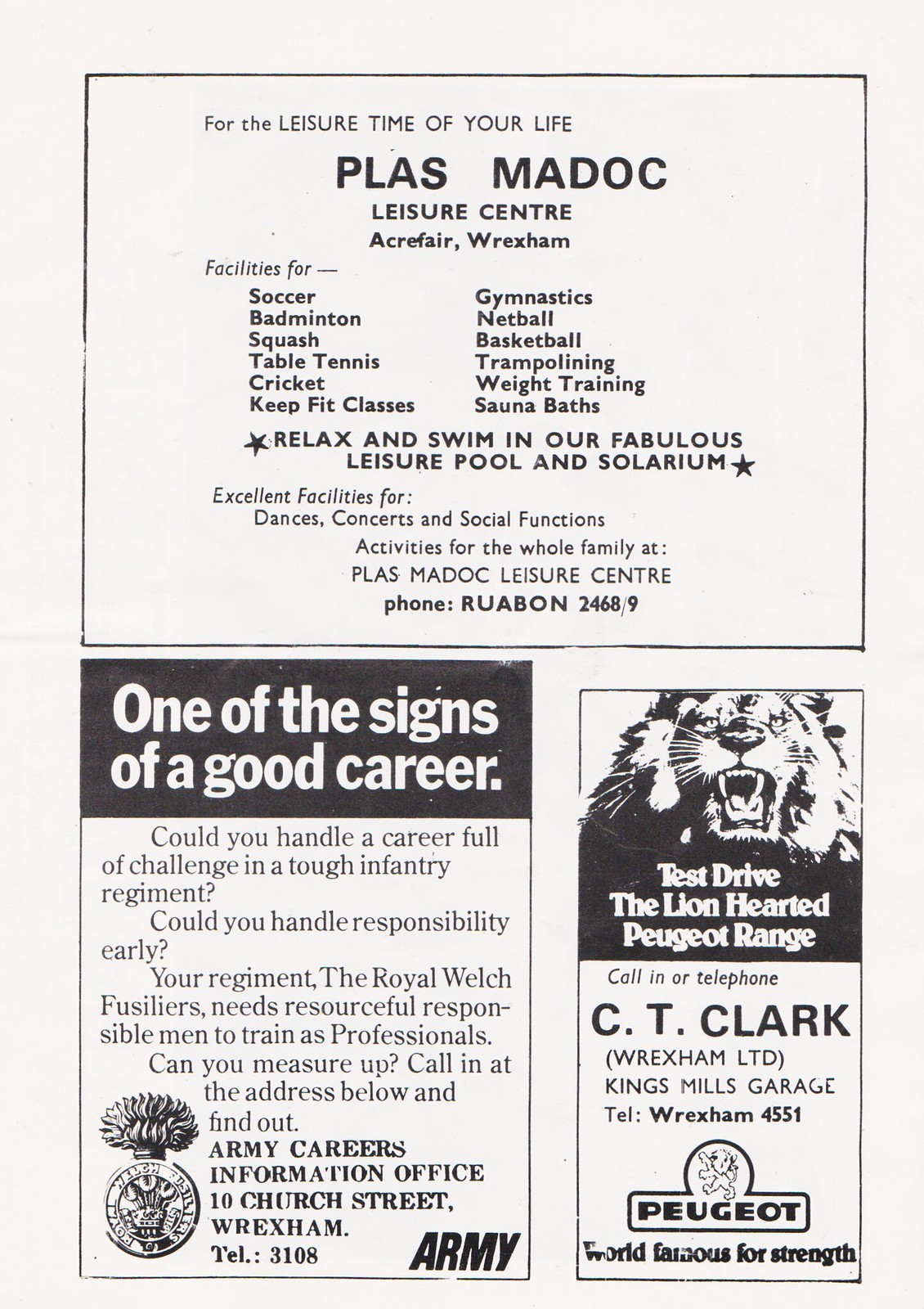This black-and-white image is a scan of an advertisement page from a newspaper or magazine featuring three distinct ads. The top half promotes the PLOS Modoc Leisure Center in Acre Fair, Wrexham, highlighting its extensive facilities, which include soccer, badminton, squash, table tennis, cricket, keep fit classes, gymnastics, netball, basketball, trampolining, weight training, sauna baths, and a leisure pool with a solarium. The center offers activities for the whole family and is an ideal venue for dances, concerts, and social functions, with a contact number provided for more details.

The bottom left ad is a recruitment notice for the Army, particularly the Royal Welch Fusiliers, emphasizing the challenge and responsibility of a career in this tough infantry regiment. It encourages resourceful and responsible men to visit the Army Careers Information Office at 10 Church Street, Wrexham, or to call for more information. The ad, with a black background and white print, is accompanied by the Army logo.

In the bottom right, an advertisement for the Peugeot automobile range features a roaring lion's head with the caption, "Test Drive the Lionhearted Peugeot Range." It invites potential customers to visit or call CT Clark, Wrexham Limited, at Kings Mills Garage. The ad underscores Peugeot's reputation with the slogan, "World Famous for Strength," alongside the Peugeot logo.